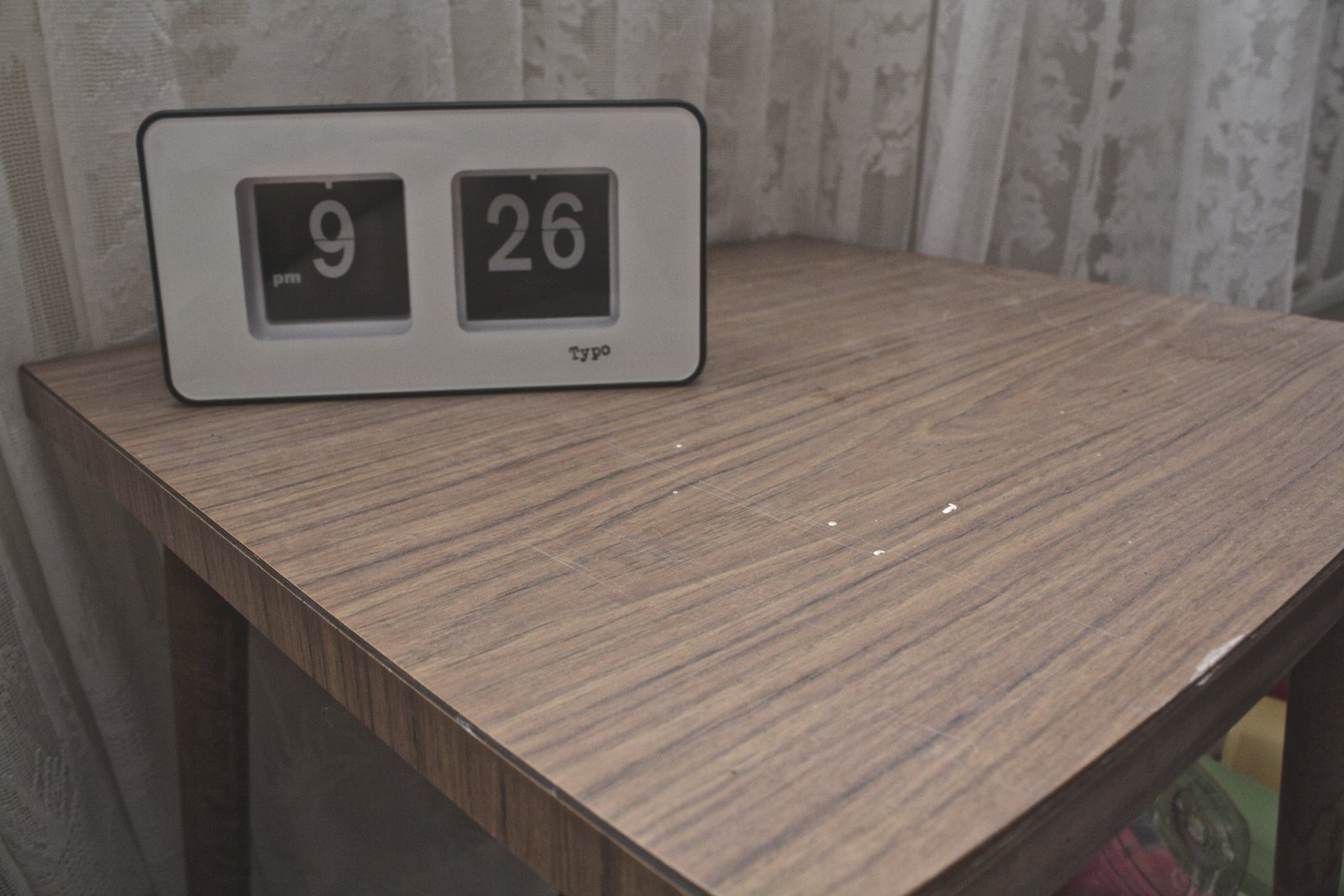The image depicts an indoor scene, possibly within a home, mostly focusing on an aged and slightly battered small side table, likely made of wood veneer or particle board. Positioned in the foreground, the tabletop is marred with signs of wear, including chipped sections revealing its non-wooden composition and a thin layer of dust. Resting atop this table is a distinctive, modern style digital clock with a white frame and black edges. The clock, which reads 9:26, has a horizontal, rectangular shape with rounded corners, and features two black square displays showing white numbers. Positioned beneath these displays is the brand name, 'TYPO,' presented in a typewriter-like font. This clock design appears reminiscent of a vintage flip clock from the early 80s. The table’s legs are brown, and a glass jar is partially visible underneath. In the background, white lace curtains obscure a window, further suggesting a domestic setting. The overall image is devoid of people and other textual elements, and though the clock reads 9:26pm, the room itself seems to be captured during daytime.